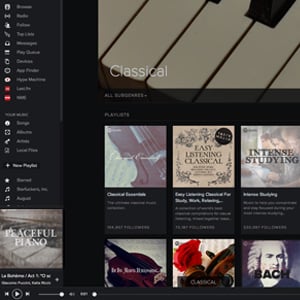This is a screenshot from a music listening app displaying various classical music playlists and albums. The left side of the screen features a vertical menu, though the text is too small and blurry to decipher. At the bottom of this menu, there is a CD cover art titled "Peaceful Piano," suggesting a collection of calming piano pieces. To the right, prominently displayed at the top, is a close-up image of a piano keyboard with "Classical" written at the bottom left, indicating the genre.

Beneath the main image, there are two rows of album covers. The first row includes three albums: one with a close-up of a violin, another labeled "Easy Listening Classical," and the third titled "Intense Studying." The second row contains another three albums: one depicting a violin, another showing the neck of a violin with a red flower, and the last featuring a portrait of the composer Bach with the word "Bach" emblazoned across it.

There are no animals, plants, trees, buildings, automobiles, airplanes, or boats in this image. The entire focus is on the music-themed graphical elements and album covers.